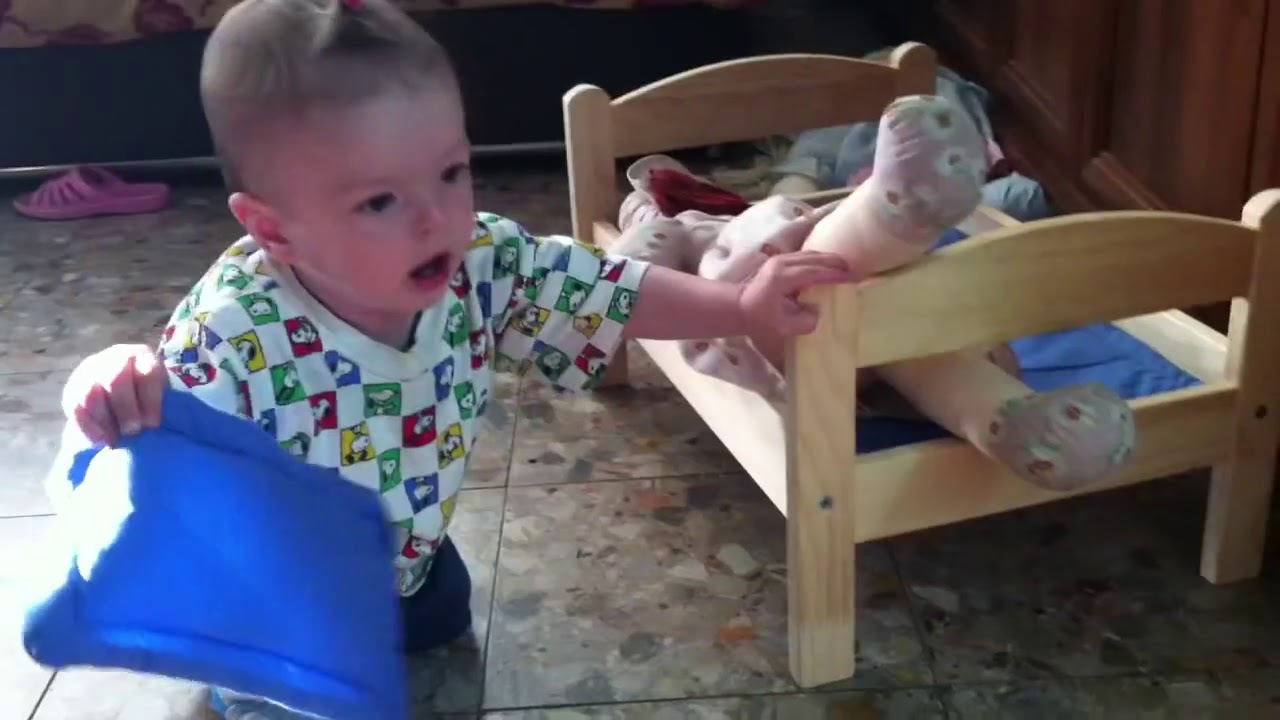In this indoor image, a toddler, approximately one year old, is playing on a tiled floor with a distinctive abstract design in shades of gray, brown, tan, and rust. The child, with short, light brown hair styled in a slight spike, is dressed in a white shirt adorned with colorful chain-link squares featuring red, green, yellow, and blue Snoopy characters. The toddler's mouth is open as if speaking, and he is holding a small, royal blue rectangular toy or pillow in his right hand, reflecting sunlight and displaying his fingers at the top.

Kneeling on the floor with blue pants, the child has his left hand resting on a small wooden toy bed. This bed, which is too small for the boy but sizeable for toys, has a pink stuffed animal with big brown eyes lying on it, and a blue thin mattress or bedding. The bed is positioned to his side, with its footboard towards the image's lower center. 

In the background, the scene includes dark-paneled walls and wooden cupboards. A single pink sandal is visible towards the upper left part of the image, slightly behind the child’s right ear. The overall setting exudes a warm, homey atmosphere with a focus on the child's playful interaction with his surroundings.